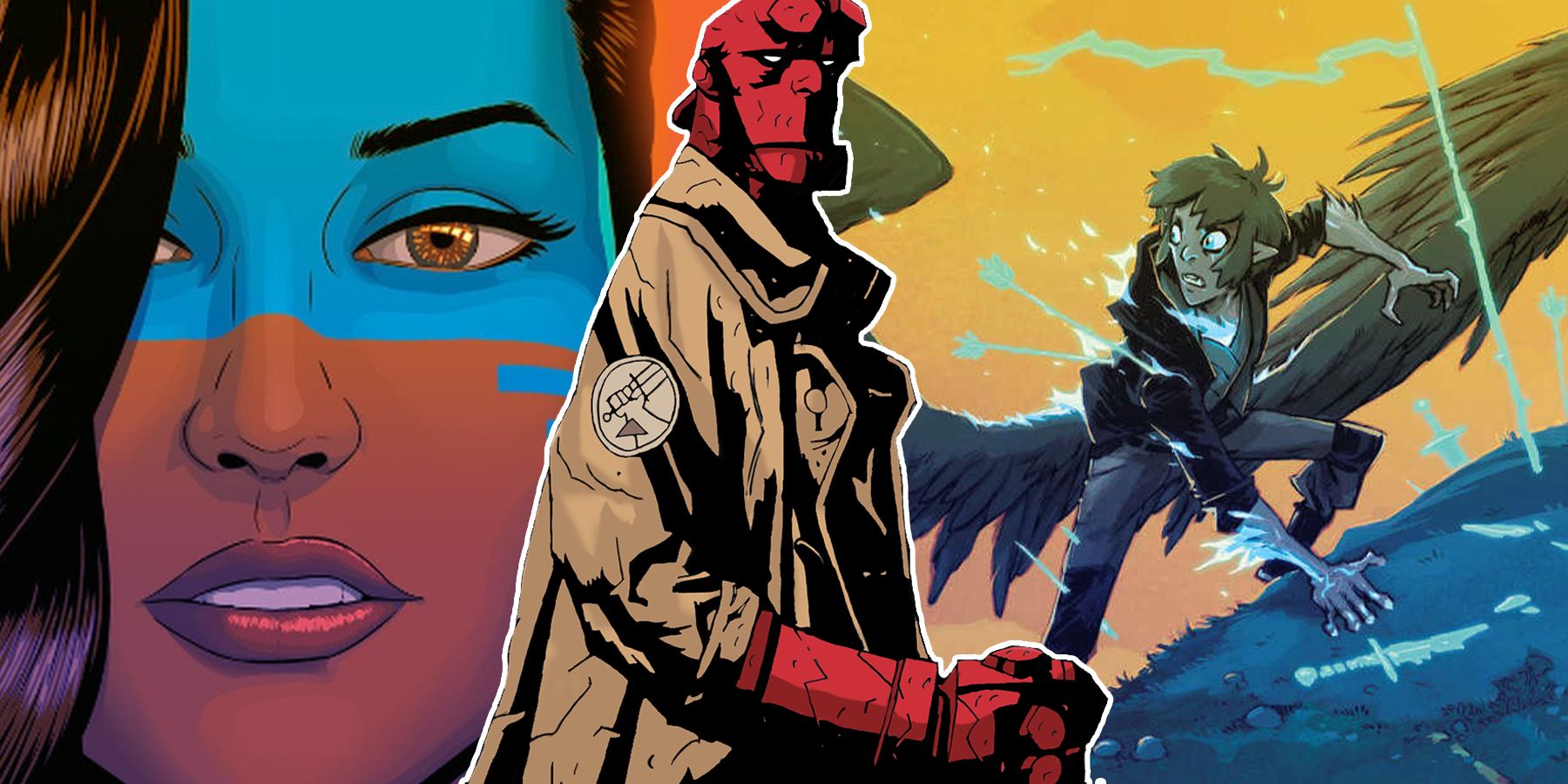In this detailed composite cartoon image, three distinct characters are illustrated against a gold background with green swirls, a darker green tree, and a blue ground. On the left, a woman with long black hair and vibrant blue face paint covering the top half of her face, coupled with two stripes on her cheek, gazes with a subtle smile. Her striking features include brown eyes, faintly visible eyebrows, brownish-red lips, and very white teeth. In the center stands a red humanoid figure resembling Hellboy, clad in a trench coat. This figure has a rugged, possibly stone-or-metal-like texture with two red protrusions on his forehead, reminiscent of horns. On the right, a creature or young man with green skin and green eyes, evoking the likeness of Beast Boy, appears terrified. His expression is one of fear as he reaches for a sword on the ground, seemingly fleeing a battle as indicated by the arrows embedded in his back. The scene sets an action-packed, intense atmosphere with all characters distinctly posed and detailed, interacting within a unified, dramatic narrative.